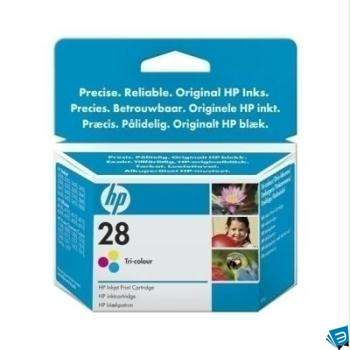The image depicts a single object centered against a white background: a color photo of HP printer ink in its original packaging. The box is primarily blue with white details and features the HP 28 tricolor inkjet print cartridge. Prominently displayed at the top, the text reads "Precise, Reliable, Original HP Inks" in white or very light blue, followed by the same phrase in two additional languages, possibly German and a Scandinavian language. Below this, the HP logo is shown above the number 28 in black letters. On the right side of the package, three photographs are depicted—a flower, a girl, and a parrot—highlighting the ink's color range. Additional information, including the cartridge's compatibility and usage details, is printed in tiny font on the package sides. The photo has a minimalist and clean presentation, likely intended for promotional use or as a stock image for sales websites.